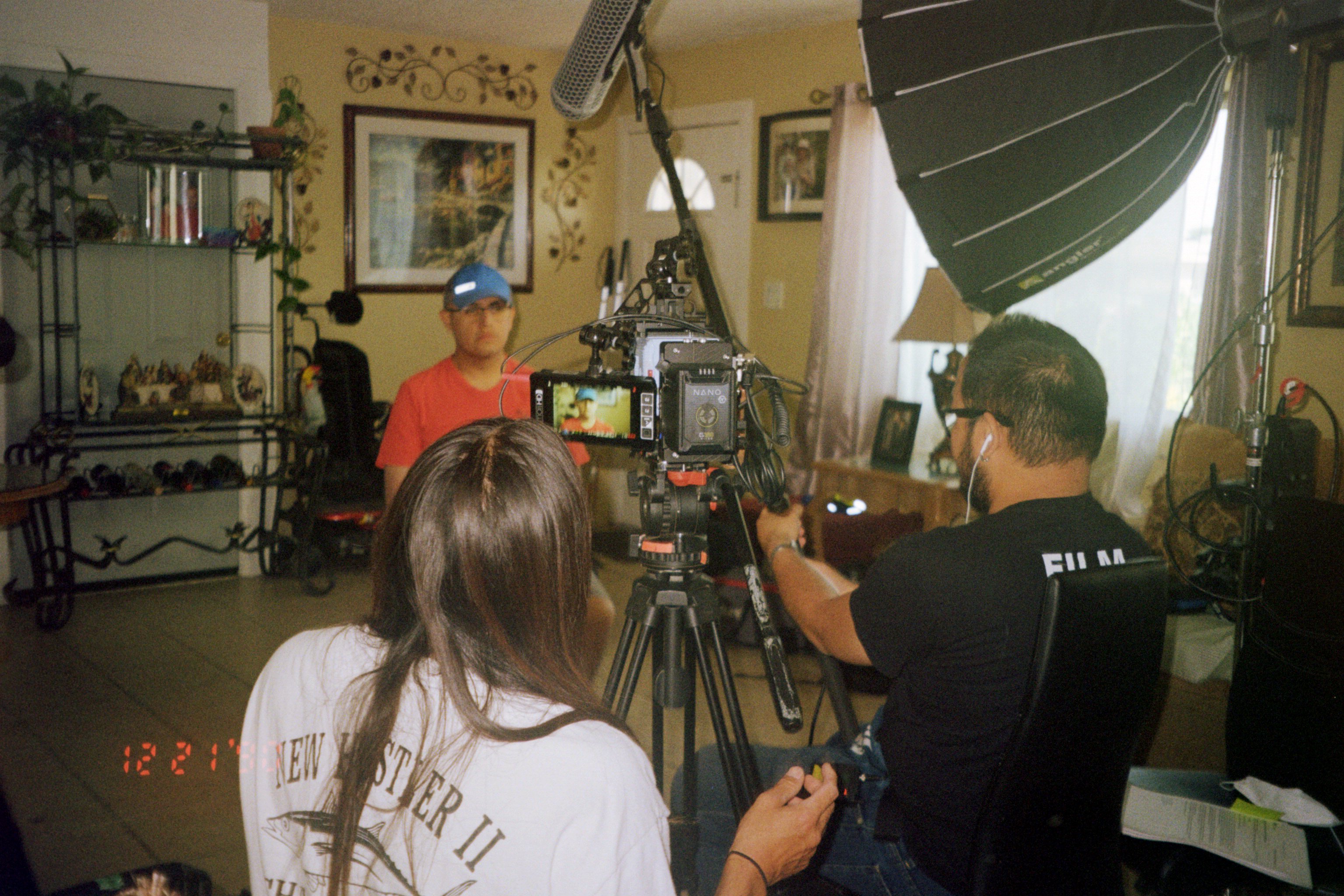In the photo, a man in a red T-shirt, blue baseball cap, and glasses sits in a chair, being interviewed for what appears to be a TV show or documentary. The scene is set in a living room, suggesting the man's home, as indicated by the presence of decorative elements such as a wire maker's rack with plants, artwork, and framed photographs on the walls. The room also includes a side table with a lamp, a picture frame, and curtains. The man is the focus of a professional film crew comprising two people. A woman with long brown hair, wearing a white T-shirt, operates the camera, while a man in a black T-shirt handles the boom microphone. Both are part of a detailed setup that includes a tripod, professional camera, and lights. The cameraman, wearing earphones, sits with his back to the viewer, while the interviewer, possibly doubling as the director, is seated across from the man being interviewed. In the background, a partial view of a date labeled "12-21" is visible, alongside some paperwork, which might be a script, hinting at the organized effort behind the production. Some ambiguity remains around a black chair that appears designed for someone with disabilities. The detailed setup and casual yet professional environment strongly indicate this is a filmed interview for a documentary or TV project.